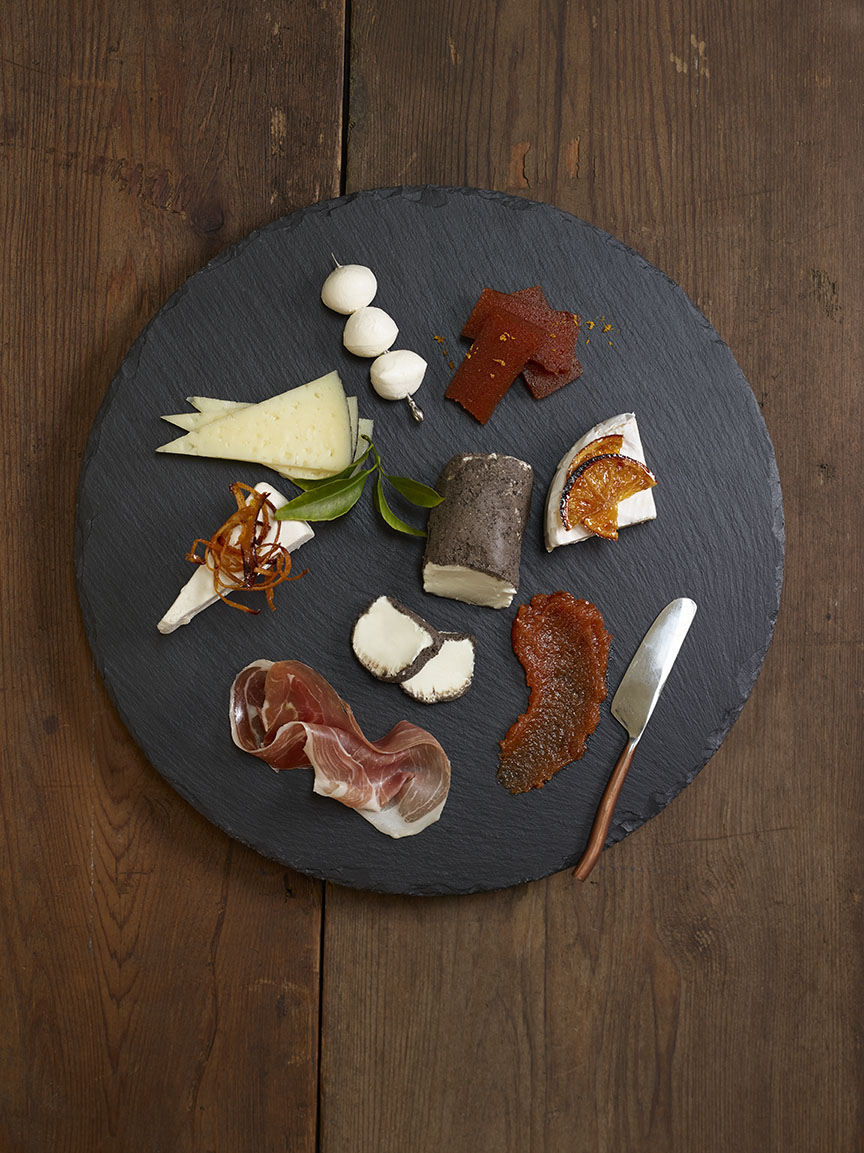The image depicts an elegantly arranged charcuterie board placed on a dark brown, wooden table, with noticeable grains and sections of the planks adding to the rustic charm. The centerpiece of the photo is a round black slate tray that almost resembles a slice of a tree trunk. This beautifully curated display features an assortment of gourmet delights. Prominently, there's a skewer piercing three small mozzarella balls, thin slices of prosciutto, and a slice of brie garnished with a dried orange slice. Also included are slices of gorgonzola, Induja sausage with a silver cheese knife boasting a wooden handle, along with several other cheese varieties and a selection of accoutrements like fruit leather and possibly fig jam. A small spreading knife suggests the presence of a spread, possibly a jam or cheese-based spread. Sprigs of rosemary add a final touch of sophistication to this inviting setup, perfect for entertaining guests or enjoying with a glass of wine.